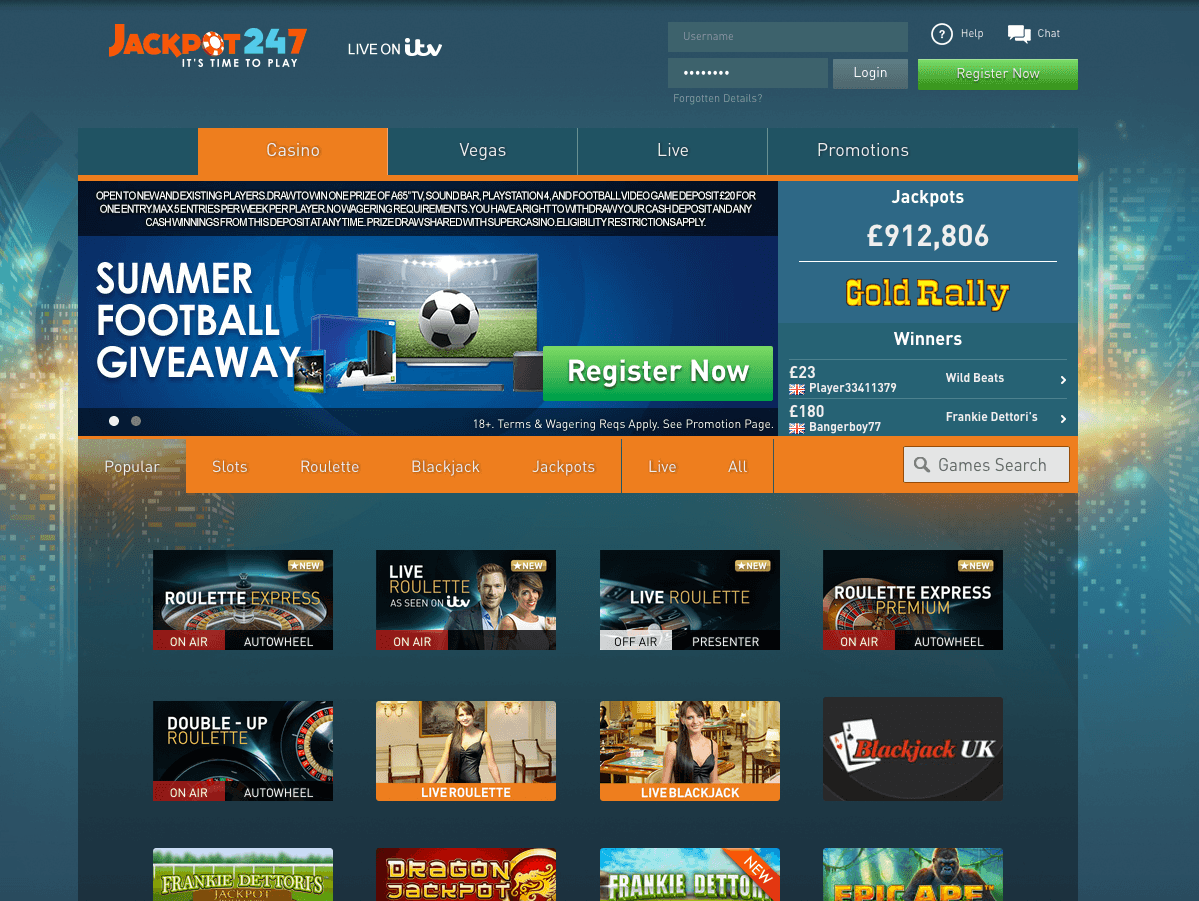The background of the image features a gradient of colors starting with a peculiar green shade, transitioning to a lighter teal, then orange, followed by yellow, returning to orange, and finally back to the teal hue. In the upper left-hand corner, the word "jackpot" is prominently displayed in orange text. Adjacent to it, "2-4" is written in blue, followed by the number "7" in orange. Below these, the phrase "time to play" is inscribed in white, alongside the phrase "live on ITV."

Beneath this section, there are several tabs. The first tab is orange and labeled "casino" in white text, while the subsequent tabs are teal, with labels reading "Vegas live" and "promotions" in white text. The lower portion of the background is black, featuring detailed information about a promotion: 

"Open to new and existing players, enter for a chance to win a prize package that includes a 65-inch TV, soundbar, PlayStation 4, and a football game. Deposit $20 for one entry with a maximum of five entries per week per player. There are no wagering requirements, and you have the right to withdraw your deposit and any winnings from the deposit at any time. Prize draw is shared with Super Casino, and visibility restrictions apply. Additionally, there is an invitation to participate in a board giveaway."

The layout of the image is carefully organized, with a vibrant color scheme and clear segmentation for information about the promotional offer.